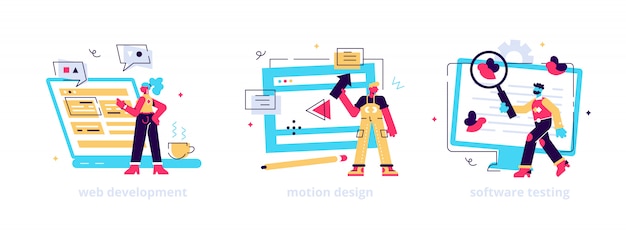The image is an animated, colorful drawing divided into three sections, each depicting a different aspect of the software and web development process, highlighting web development, motion design, and software testing. 

On the left, labeled "Web Development," there is a tiny woman with blue hair, dressed in a yellow tank top, jeans, and pink high heels. She stands beside an oversized laptop, actively designing a web page. The web page features various icons and bubbles, though it lacks written content. Beside her on the desk, there's a cup of steaming coffee or tea, adding a cozy touch to the workspace.

In the center, labeled "Motion Design," a man is shown manipulating symbols and templates on a large tablet screen. He wears gold overalls over a black t-shirt, matching gold sneakers, and a gold cap tilted slightly to his left. Around him, a giant pencil lies on the ground, emphasizing the creative nature of his task.

On the right, labeled "Software Testing," another man stands in front of a desktop computer. He has blue hair, a beard, and is dressed in a pink shirt with yellow sleeves, purple pants, and pink shoes. He holds a giant magnifying glass, symbolizing his role in meticulously examining the web page for errors. All the computers featured in the drawing are blue with orange writing, and the characters have a distinctive pink-red skin tone.